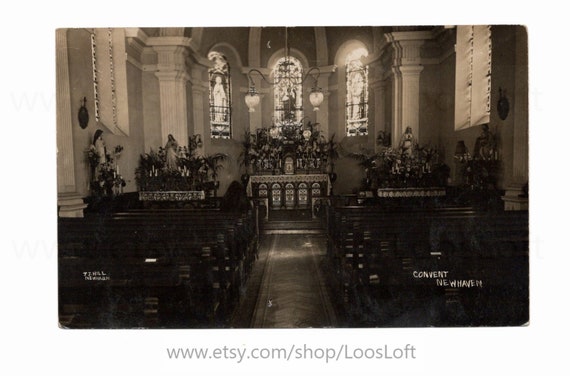This evocative sepia-toned photograph captures the solemn interior of a historic church, possibly Catholic or Lutheran. The image, taken from the midpoint of the sanctuary, reveals a series of seven to eight rows of classic wooden pews flanking a central aisle, with a lone figure seated in the front row. The expansive, dome-shaped sanctuary features sizable stained-glass windows along its far side, adding a touch of grandeur. At the forefront lies a large, prominent altar flanked by what appear to be small shrines or niches holding statues, likely depicting Jesus Christ and the Virgin Mary. Scattered around the front and sides are additional religious statues contributing to the sacred ambiance. Visible text at the bottom left reads "T.J. Hill," and on the lower right, it says "Covenant New Haven," suggesting a connection to the church's identity. The image appears to be available for purchase, indicated by an Etsy link, etsy.com/shop/loseloft, subtly included in the photograph.